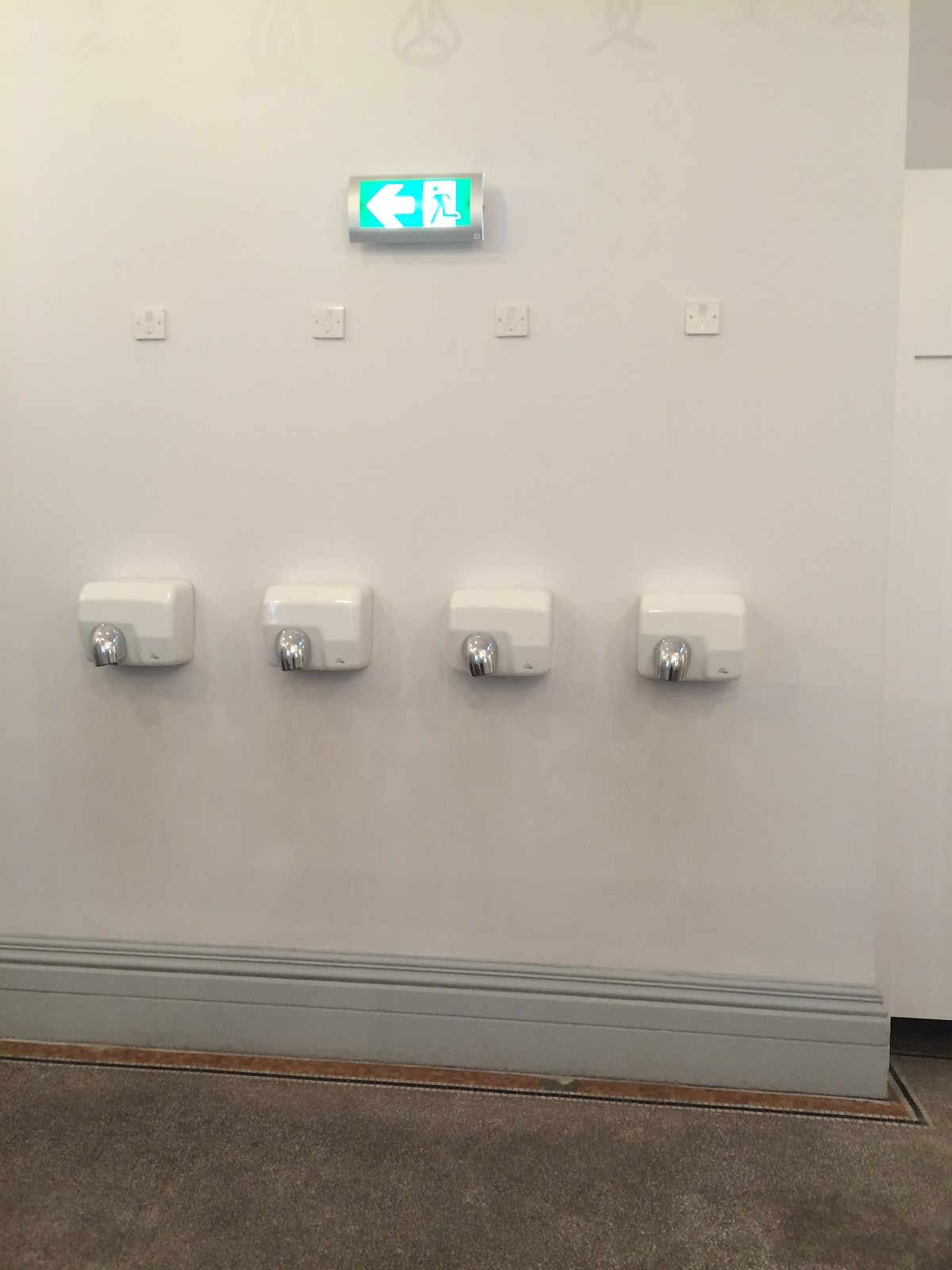The photograph captures a detailed interior scene dominated by a large white wall. Prominently, there is a rectangular, illuminated exit sign at the top of the image. This sign features a silver outline, a light turquoise background, and a white arrow pointing to the right. It also includes a small white rectangle depicting a silhouette of a person walking or running. Below this sign, the wall displays four equally spaced square panels that appear to be light switches or outlets. Along the lower portion of the wall, four white hand dryers are neatly lined up in a row. Each dryer has a silver nozzle directed downward. The wall is trimmed with a light gray wooden border towards the floor, which is dark brown and shows some signs of wear. The scene hints at the possibility of another room to the right, marked by additional white wall space with a gray top border.